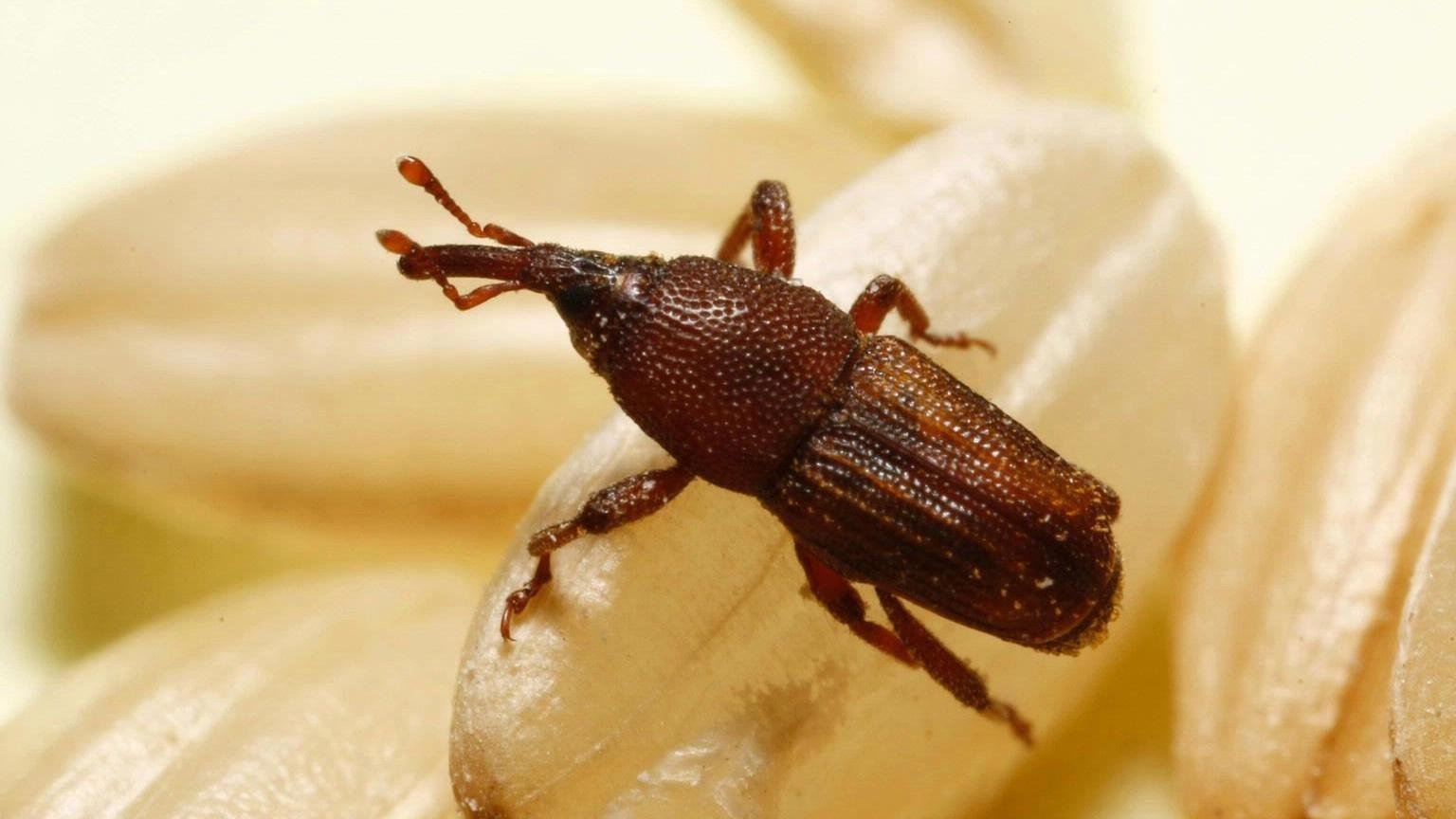This image showcases a close-up, photographic capture of a reddish-brown insect, possibly a beetle, positioned diagonally from the bottom right to the top left. The insect features a long, tapered snout, six legs, two antennas, and a rounded posterior. It has a bumpy, almost dotted surface, giving it a slightly slimy or moist appearance. The insect is perched on what appears to be a light brown, oval-shaped grain, likely an oat, reflecting light from a camera flash. This oat is surrounded by at least four or five others, all beige and cream-colored, creating a neutral background that is out of focus, emphasizing the detailed texture and coloring of the insect. The setting appears to be indoors, enhancing the clarity and detail of the insect and the grains.